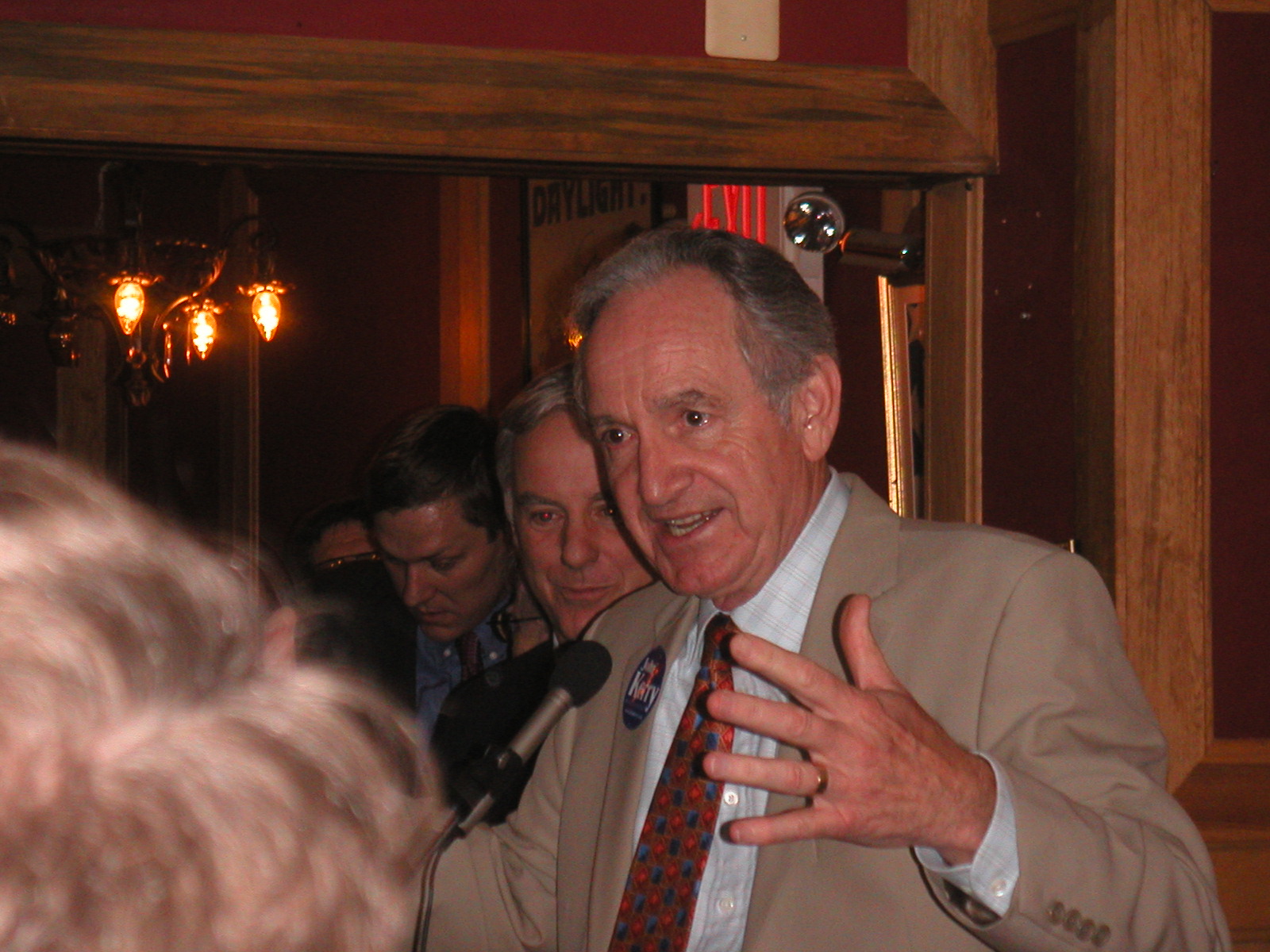In the image, an older gentleman stands at a casual speaking event, holding a microphone. He is dressed in a camel-colored suit jacket and a white dress shirt that features subtle, light gray stripes. His tie sports a red and blue checkered pattern. On the right side of his chest, he wears a circular, blue political pin, which might say "Cary." The event appears to be set inside a restaurant, characterized by wooden-framed entryways around the speaker. Behind him, two other men are seen looking downward, seemingly focused on something else. Additionally, part of another person can be seen in front of him, with only their hair visible. There is also a sign positioned above and behind to the left of the speaker.